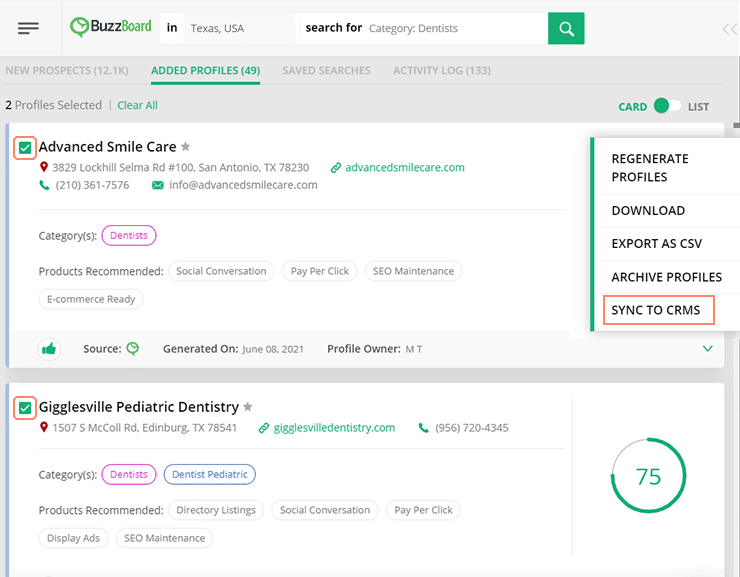The image showcases a website interface set against a gray background. In the upper left corner, there is a black "more options" button symbolized by three horizontal lines. Adjacent to it is a green speech bubble icon with the text "BuzzBoard" where "BUZZ" is in black and "BOARD" in green. Below it, "In Texas, USA" is displayed along with a search bar pre-filled with "search for category dentists" and a green search icon.

The main content features several statistics including "New Prospects: 12.1k," "Added Profiles: 49" (which is underlined in green), "Save Searches," and "Activity Log: 133." There's also an option indicating "Two profiles selected" with a "Clear All" button next to it.

The first profile listed is "Advanced Smile Care," highlighted with a green checkbox within a red-outlined box. This entry includes the address "3829 Lock Hill-Selma Road, 100 San Antonio, Texas, 78230," the website "advancedsmilecare.com," the phone number "210-361-7576," and the email "info@advancedsmilecare.com." The profile is categorized under "Dentists" and lists recommended products such as "Social Conversation," "Pay-Per-Click," "SEO Maintenance," and "E-commerce Ready."

The second profile, "Gigglesville Pediatric Dentistry," also highlighted by a green checkbox within a red-outlined box, lists the address "1507 South McColl Road, Edinburgh, Texas, 78541," and is classified under "Dentists" and "Dentists Pediatric." The recommended products for this practice include "Directory Listing," "Social Conversation," "Pay-Per-Click," "Display Ads," and "SEO Maintenance." A green circle with the number "75" is displayed on the right side of this profile.